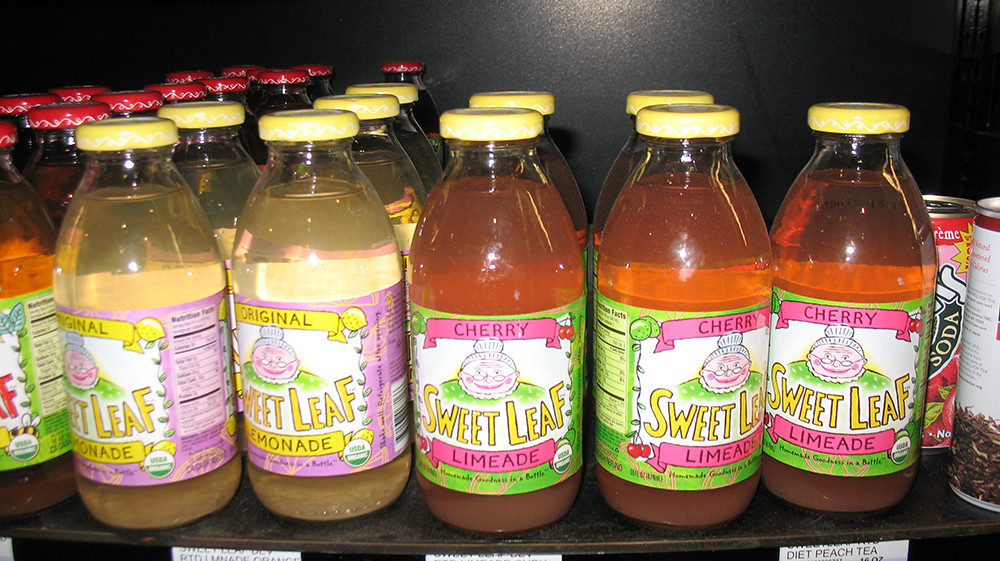This is a photograph of a store shelf filled with various beverages. Prominently displayed are Sweet Leaf brand drinks in glass bottles with yellow caps. In the center-left, there are two rows of the Original Sweet Leaf Lemonade, identifiable by its light yellow liquid and a cartoon granny on a purple background. This lemonade label also indicates "USDA Organic" in a small label on the bottom right corner. To the right of the lemonade, there are three rows of Sweet Leaf Cherry Limeade, characterized by its orangish liquid and green background with the same cartoon granny. On the far left, there's another Sweet Leaf beverage with an orangish liquid, but the label is not fully visible. On the far right, there are some canned drinks, and a price tag indicating "diet peach tea" is partially visible on the shelf below. The shelf itself is dark, possibly black or brown, providing a contrast to the vibrant bottle labels.